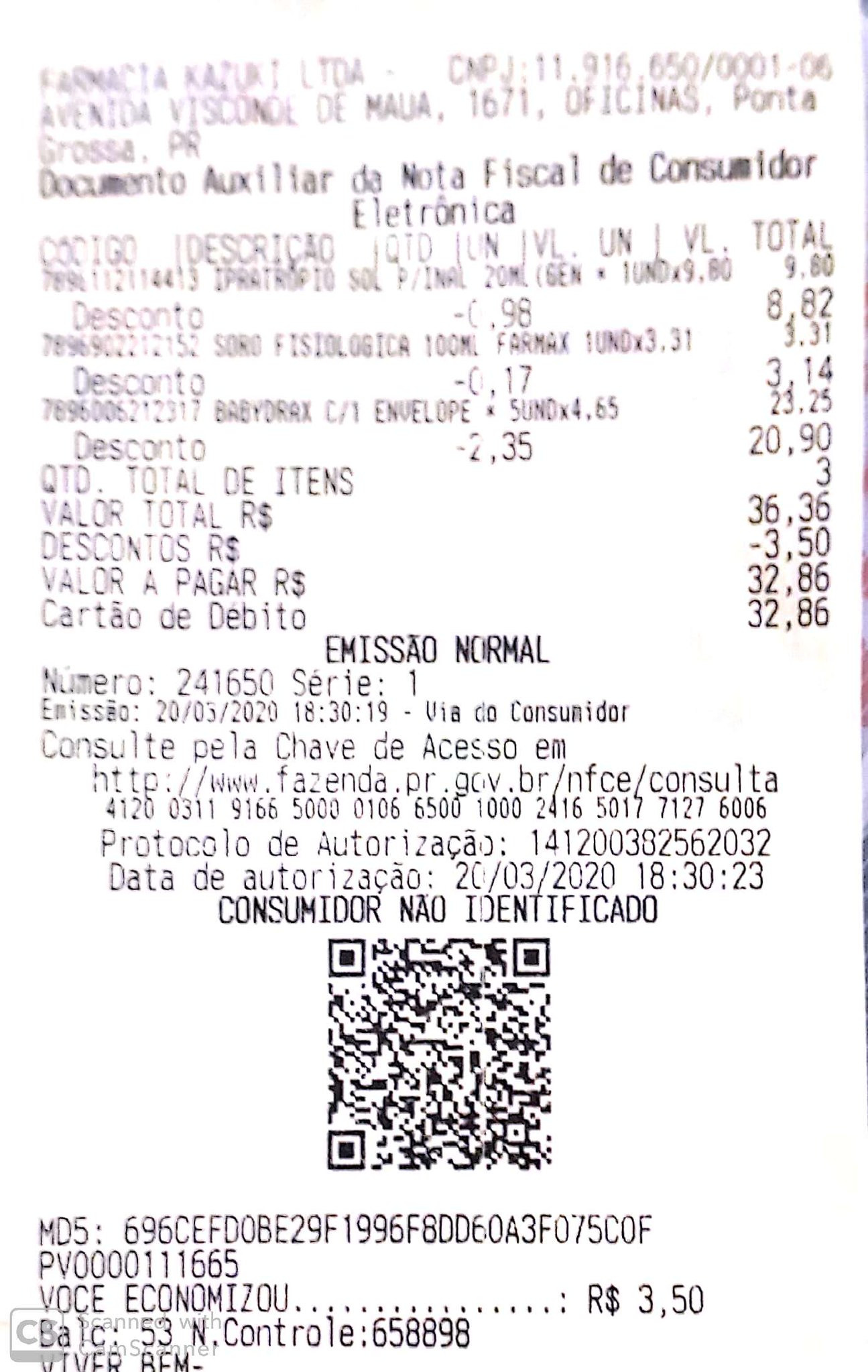The image depicts a vertically rectangular, white receipt with black writing, printed from a store. The receipt appears to be in Portuguese, indicated by phrases like "Documento Auxiliar de Nota Fiscal de Consumidor Eletrônica" at the top. Details include itemized purchases, quantities, and discounts with entries such as "Codio Descriptio 980," "Descanto 882," "Descanto 314," and "Descanto 2090." The total quantity of items is 3, with a total value (Valor total) of R$36.36, discounts (Descantos) amounting to R$3.50, and the amount to be paid (Valor a Pagar) listed as R$32.86, paid via Debit Card (Cartão de Débito). The transaction date is noted as March 20, 2020 (2003-2020) with a time stamp of 18:30:19. At the bottom of the receipt, there is a QR code and a website URL: http://www.fazenda.pr.gov.br/nfce/consulta, suggesting it can be used for further information or verification. Numerous serial numbers are also present at various points across the receipt.